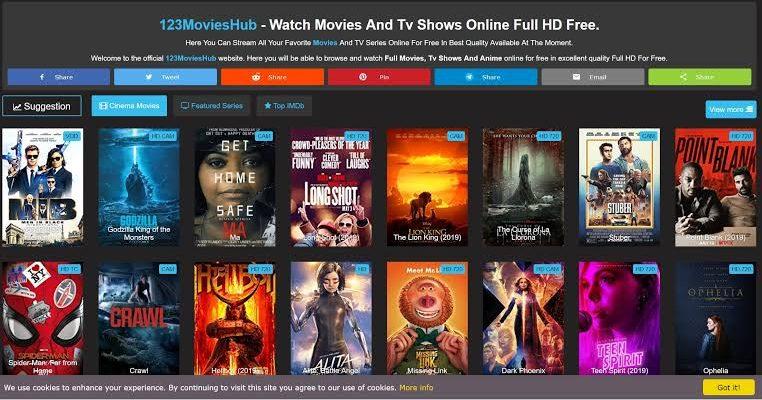This screen capture depicts the homepage of a movie streaming website named "123 Movies Hub." At the very top, the site's name is prominently displayed in a combination of blue and white text. Below the title, a tagline reads, "Watch movies and TV shows online in full HD for free," emphasizing that users can stream their favorite content at the highest quality available.

Immediately beneath this tagline, a welcoming message is displayed: "Welcome to the official 123 Movies Hub website. Here you can stream all your favorite movies, TV series, and anime online for free in excellent HD quality." This message encourages visitors to browse the site's extensive collection of entertainment options.

Under this message, a row of social media sharing buttons is clearly visible. The buttons include a blue "Facebook share," a blue and white "Tweet," an orange and white "Reddit share," a red and white "Pinterest pin," another blue and white sharing option, a gray and white "Email" button, and a green and white "Share" button.

Following the social media buttons are several submenu options in gray and white. These include "Suggestions," "Cinema Movies," "Featured Series," and "Top IMDb." To the right, a "View More" button prompts users to explore additional content.

The main body of the screen is filled with a colorful array of movie posters. Titles displayed include recent releases such as "Men in Black," "Godzilla," "Maw," "Long Shot," Disney's 2019 remake of "The Lion King," "Stuber," "Point Blank," "Spider-Man: Far From Home," "Crawl," "Hellboy," "Alita: Battle Angel," "Missing Link," "Dark Phoenix," "Teen Spirit," and "Ophelia." Each poster has a small blue box with black font in the corner, providing additional information.

At the bottom of the screen, a gray bar states, "We use cookies to enhance your experience. By continuing to visit this site you agree to our use of cookies." An orange "More Info" button and a gold "Got It" box are available for users to manage their cookie preferences.

The movie posters showcase a variety of vibrant colors including shades of white, blue, black, red, orange, gray, burgundy, gold, purple, pink, and more, adding a visually appealing diversity to the page.